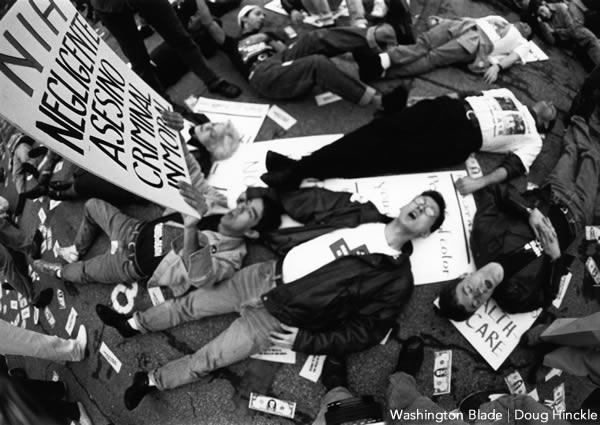This iconic black and white photograph captures a moment of a lay-down protest with numerous individuals lying face-down on the pavement, amidst handmade signs and scattered fake dollar bills. The text at the bottom right corner credits the photographer, Doug Hinkle, and identifies the image as published in the Washington Blade. The scene is somewhat blurry yet vividly depicts various protestors, possibly both men and women, appearing in different languages, with some signs specifically calling out negligence, criminality, and immorality, particularly in reference to the healthcare system and the National Institutes of Health. The participants, dressed in casual outfits like dungarees and t-shirts, seem unified in their chant or message, highlighting an impactful moment of activism likely tied to a significant historical movement.